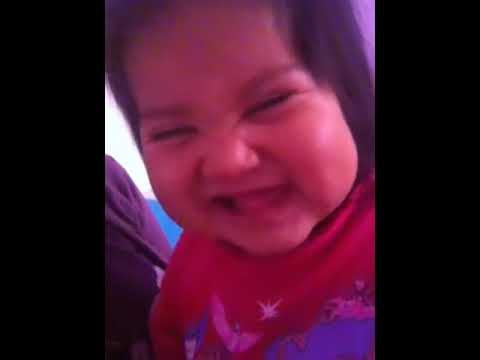This close-up photo captures a young toddler, likely one or two years old, with black, wispy hair that reaches down to their shoulders. The child has darker skin and deep brown eyes, with thin black eyebrows. The baby’s lips are tightly closed, yet subtly curled into a smirking, mischievous smile as they gaze slightly downward. Dressed in a red shirt adorned with fairy-tale characters, including castles, birds, and fairies, the child exudes a certain charm. The setting includes purple elements on the left, possibly an armrest, and blue bedsheets with white clouds in the background. Vertical black bars frame the photo on each side, adding a touch of contrast to the scene.